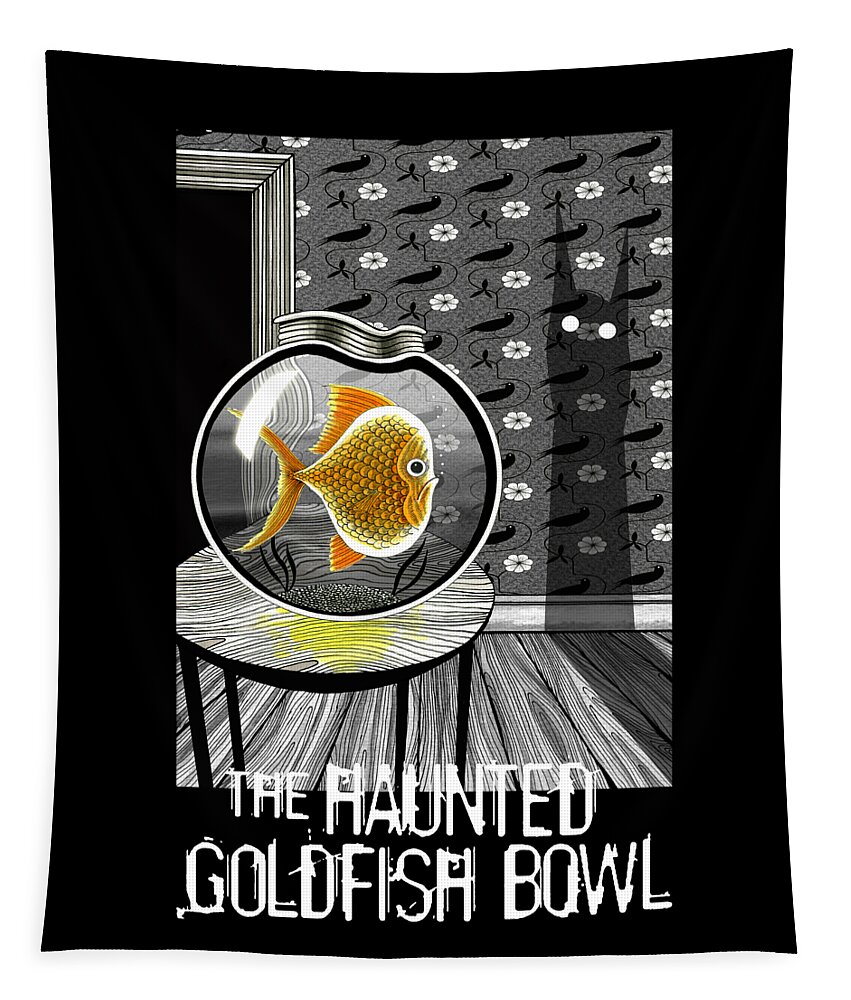This artwork, seemingly the cover of a comic or book, titled "The Haunted Goldfish Bowl" in eerie, stylized text, features a singularly colored, large orange goldfish with a displeased expression, trapped within a meticulously detailed fishbowl. The bowl rests atop a circular wooden table positioned on a hardwood floor. The background is dominated by a grayscale wallpaper that evokes a Haunted Mansion aesthetic, adorned with ravens and floral patterns in black and gray. White molding frames the open doorway leading into a pitch-black space. Adding to the spooky ambiance, a tall, lean shadow with pointed ears and glowing white eyes, resembling a ghostly bat or cat, looms ominously on the right side, hinting at the goldfish's impending danger.